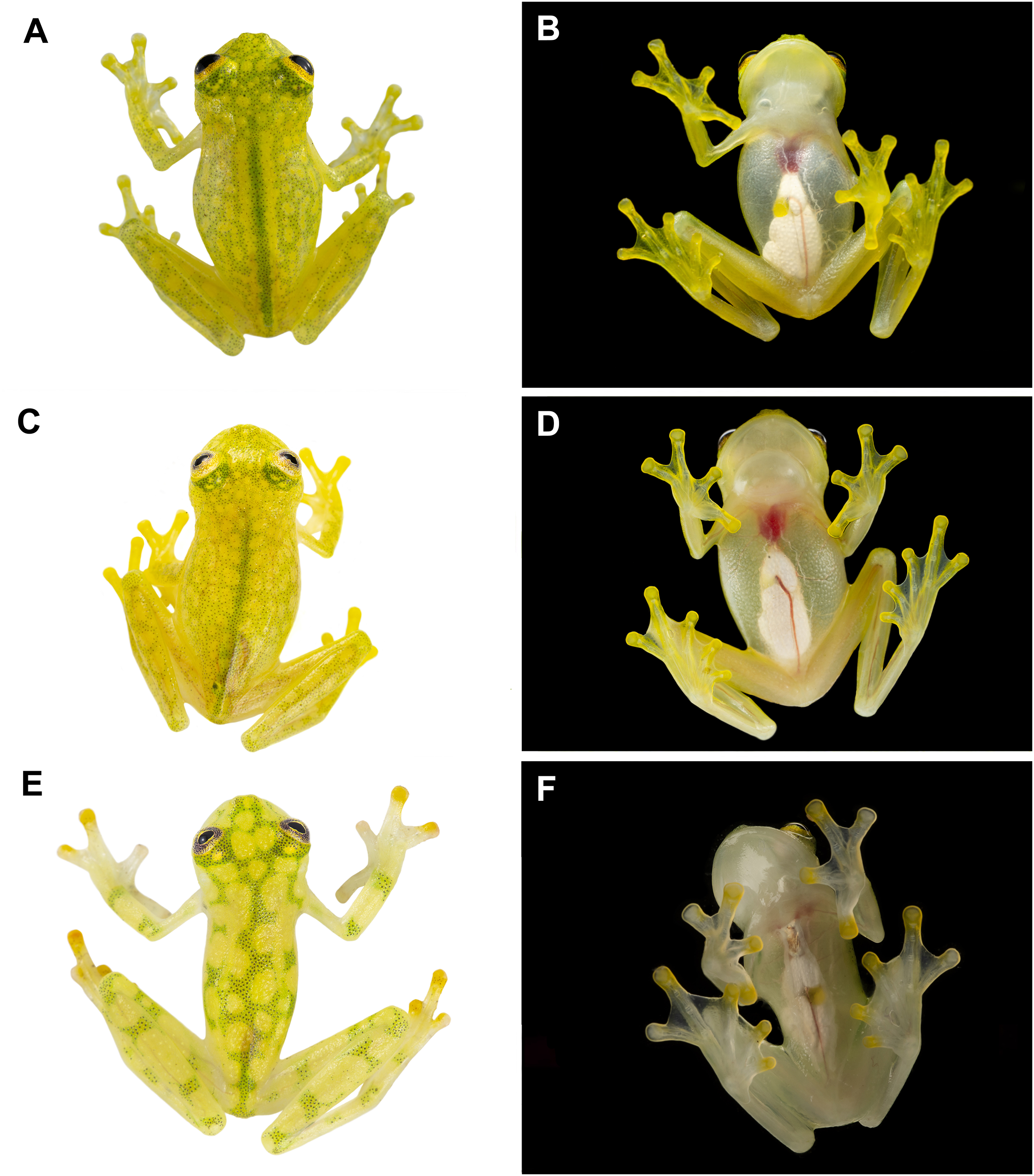The image showcases six detailed figures of a green frog, presented in a format resembling an educational prop. The figures are divided into two columns against contrasting backgrounds: the left side features images labeled A, C, and E on a white background, and the right side features images labeled B, D, and F on a black background. Each side has three perfect squares with the frog in different poses. In all six images, the frog displays a green exterior with a white, somewhat transparent belly, allowing a glimpse of its internal structure, particularly on the right side images. The frog is portrayed in varied positions, appearing to crawl with its legs splayed out. The clear and well-lit presentation enhances the visibility of the frog's anatomical details, making it a valuable visual aid for learning.